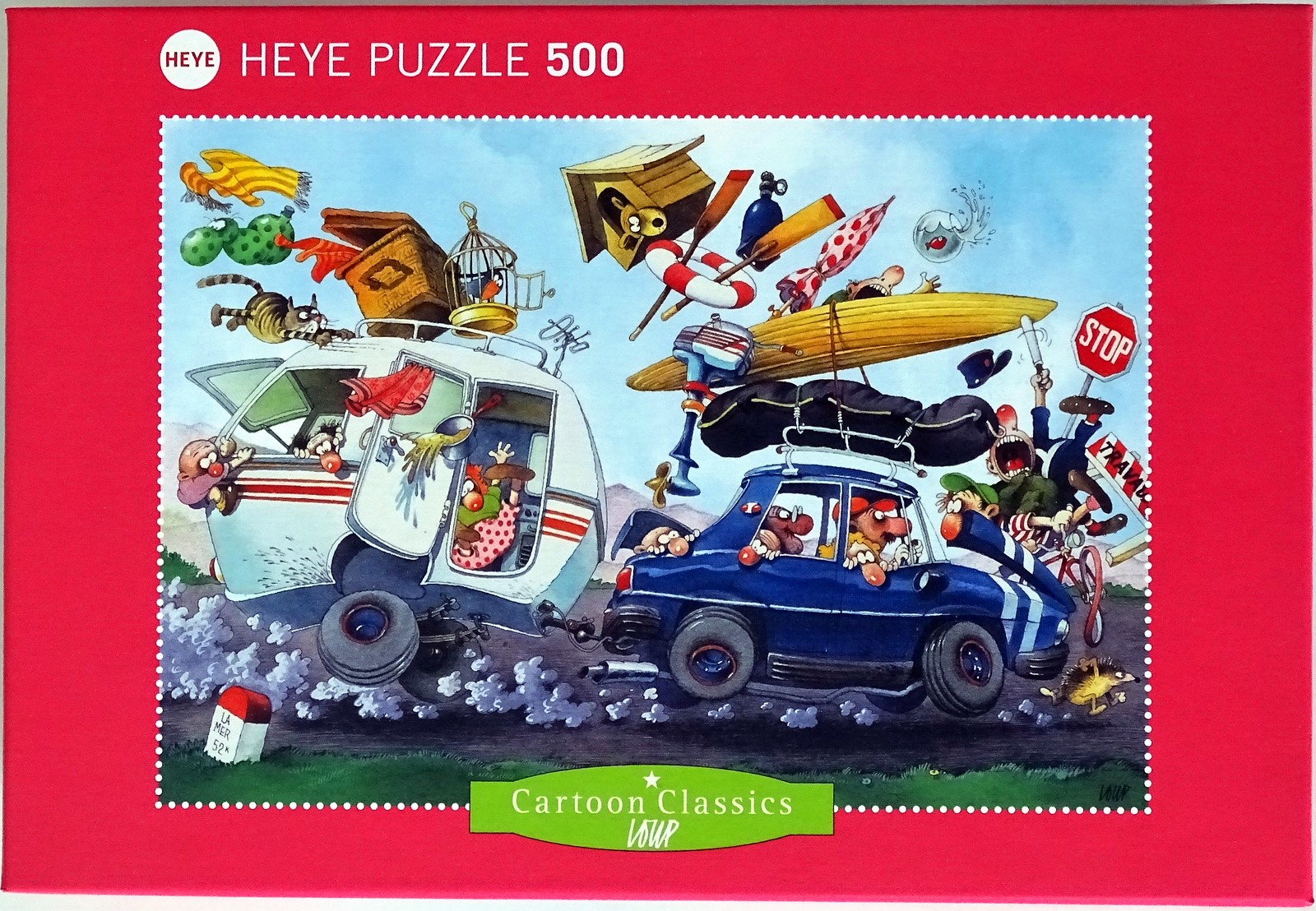The box cover of the Heye Puzzle 500 features a vibrant and detailed design framed by a thick red border. At the top center, a small white circle contains the brand name "Heye" (spelled H-E-Y-E). To its right, the text "Heye Puzzle 500" is prominently displayed, with "500" in bold white on a red background. 

The central artwork showcases a chaotic yet humorous illustration of a blue car towing a small motorhome. The scene is filled with cartoonish energy, depicting various items seemingly exploding from the vehicle. Notable objects include a canoe, a doghouse, a fishbowl, a budgie cage, an outboard motor, a life raft, oars, a tent, flying umbrellas, and baskets. The car is surrounded by a flurry of activity, including a police officer, a hedgehog outrunning the vehicle, and other whimsical characters, all rendered in an exaggerated, animated style. The air is thick with smoke, emphasizing the frenetic motion.

At the bottom of the image, a green rounded square label bears the text "Cartoon Classics" in white, with a white star inside the green box and the word "BOUP" beneath it. This detailed illustration perfectly captures the playful essence of the puzzle's design, promising an engaging and humorous assembly experience.